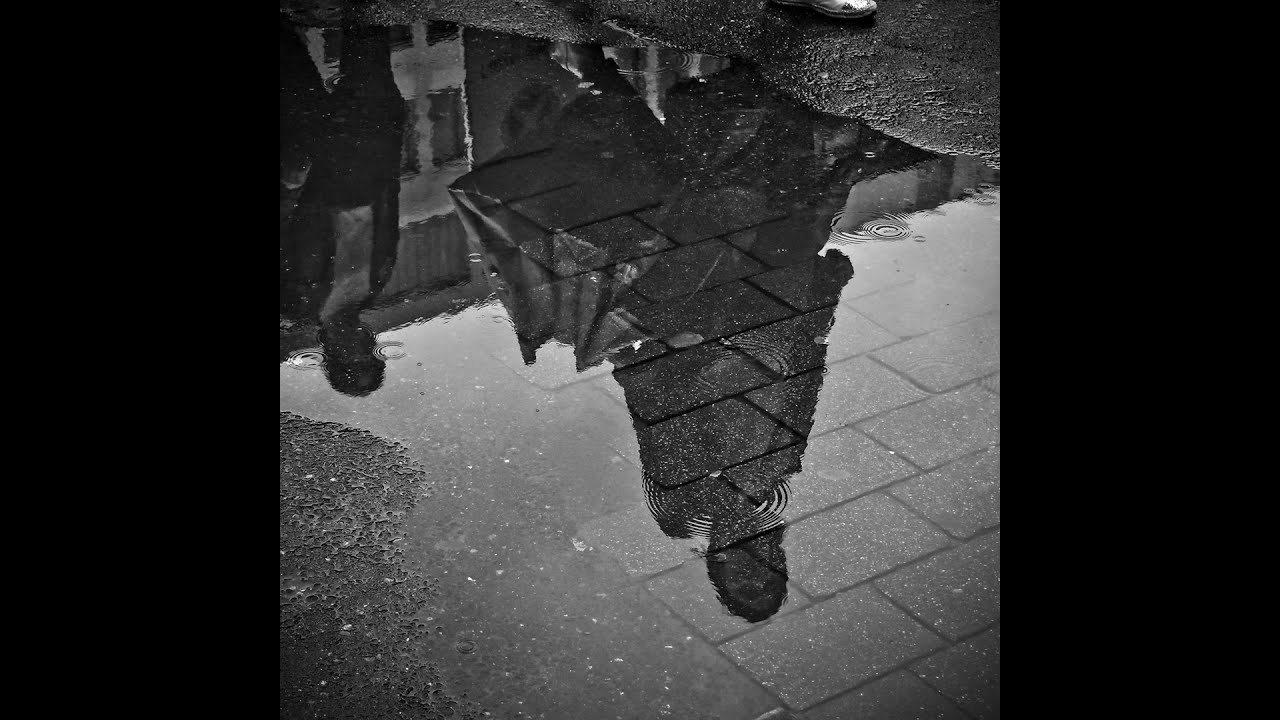The black-and-white photograph depicts a somber, rainy scene. At the center is a shallow puddle on a mixed surface of blacktop and brick pavement, occupying approximately 50% of the landscape-oriented image. Framed by black rectangles on the left and right, the puddle reflects the upside-down silhouettes of two people walking. One figure, discernible by dark clothing and a white top, stands beside a taller figure near a possible object. Ripples on the puddle's surface, created by the ongoing light rain, subtly distort the reflections and enhance the melancholy mood. In the background of the reflection, several multi-story buildings loom, adding depth to the composition. Sparse ripples indicate gentle raindrops, further highlighting the delicate ambiance of the scene.